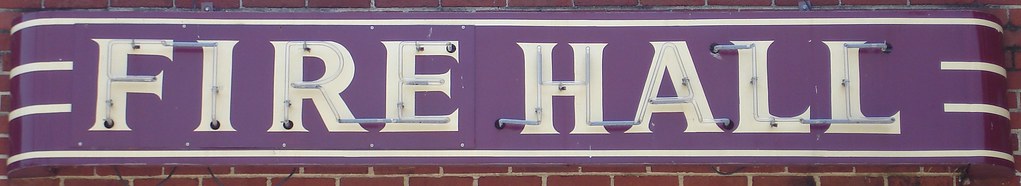The image depicts a long, horizontal outdoor sign mounted on a red brick wall with gray grout. The sign itself is purple and features large, bold white letters spelling "FIRE HALL." There is unlit neon tubing visible within the letters. The sign is bordered by thin white lines: one across the top, one across the bottom, and shorter lines on either side of the text. The sign curves inward slightly at the side edges. The photograph, taken during the daytime, shows no people, animals, plants, or vehicles, and it appears to be captured with a personal camera or a cell phone.